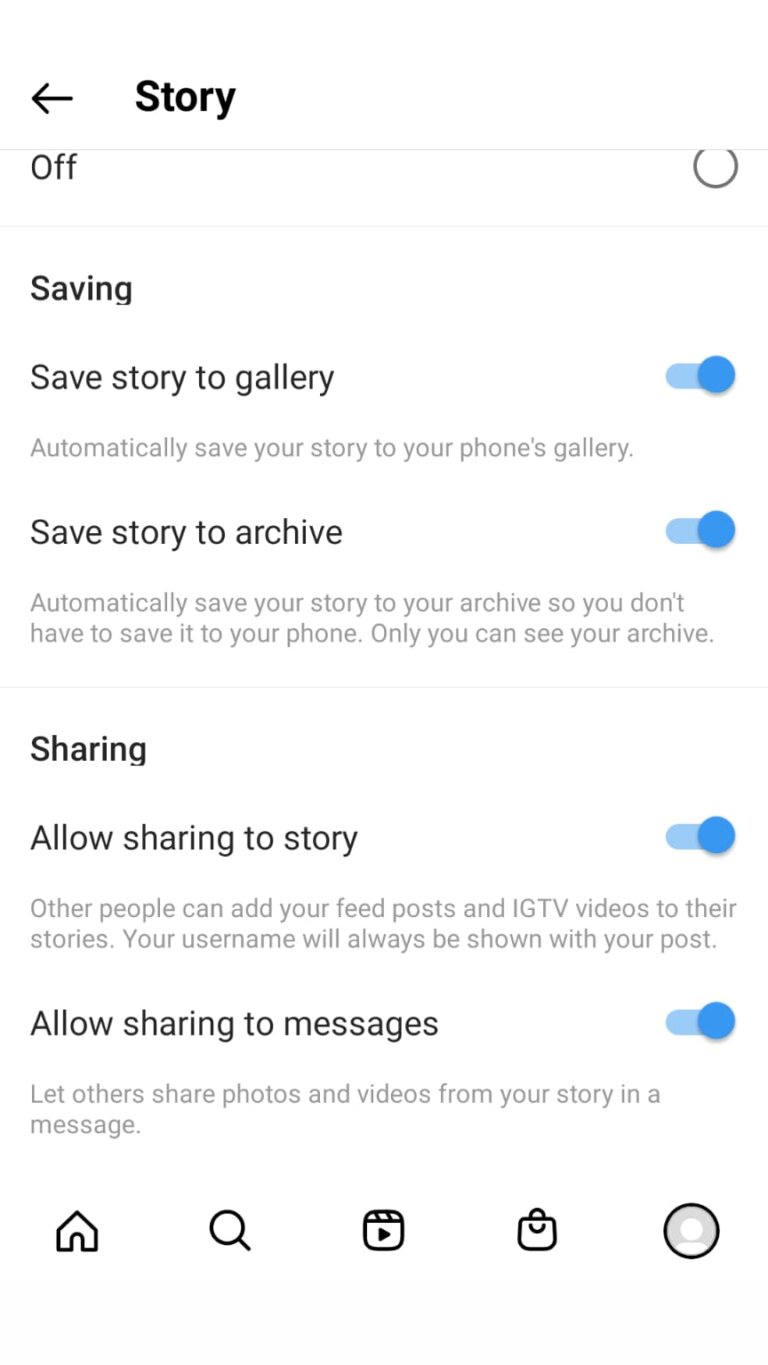The image portrays a detailed settings interface for managing story features on a social media application. In the top left corner, an arrow points left adjacent to the text label "Story." Below, a section divider indicates “Off.” There is a prominent box labeled "Saving," within which a toggle switch is activated beside the option "Save Story to Gallery." This option is further explained with text stating, "Automatically save your story to your phone's gallery."

Further down, another setting reads "Save Story to Archive," accompanied by a toggle switch. The explanatory text here notes, "Automatically save your story to your archive so you don't have to save it to your phone." Additional sections follow, including "Sharing," with two toggle options: "Allow Sharing to Story" and "Allow Sharing to Messages." The first toggle, when enabled, allows other users to add your feed posts and IGTV videos to their story, with your username appearing alongside the shared posts. The second toggle permits others to share your story's photos and videos in personal messages.

At the bottom of the interface, icons represent different app functions: a house, a magnifying glass, a square with a play button inside, and a shopping bag with handles on the side and top. Lastly, a circular icon, resembling an avatar, is detailed along with dividing lines, contributing to the interface's organized visual structure.